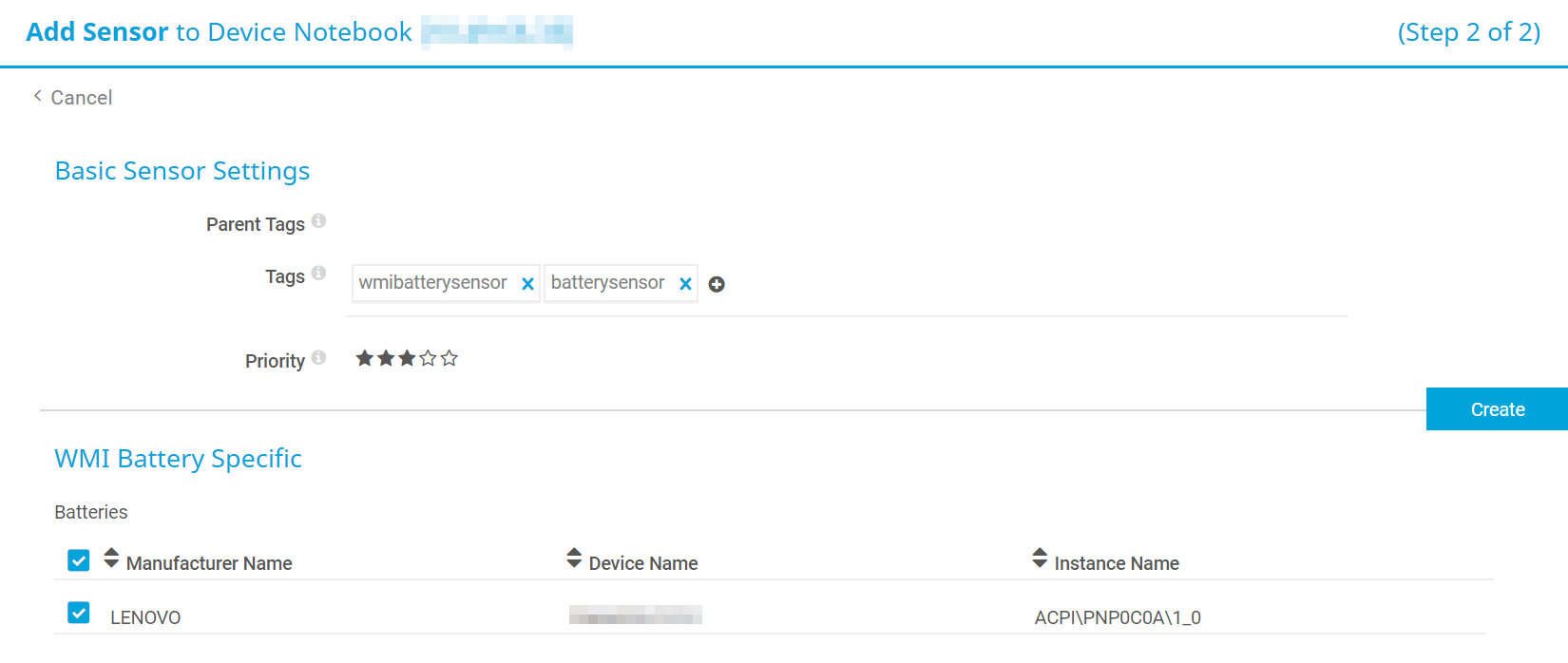This image is a detailed screenshot of a software menu with a predominantly white background. At the very top left, in blue text, it reads "Add Sensor to Device Notebook." Adjacent to this, there's pixelated and blurred text, with "Add Sensor" highlighted in bold. On the top right, it states "(Step 2 of 2)." A long, thin, horizontal blue bar extends across the screen from left to right, beneath this header.

On the left side, there is a "Back" button labeled as "Cancel." Directly below this, in blue text, it reads "Basic Sensor Settings." Following this, there is an option for "Parent Tags" accompanied by an informational icon. The selected tags are displayed as "WMI Battery Sensor" and "Battery Sensor," each with an option to remove them (indicated by an "X").

Further down, "Priority" is indicated with a set of five stars; the first three stars on the left are gray, while the two on the right are white with a gray border. Below this, a long thin gray line stretches across the screen, ending in a blue rectangular button labeled "Create" in white text.

In the subsequent section, titled "WMI Battery Specific" in blue text on the left, it lists specific attributes about the battery. It includes fields for "Manufacturer Name," "Device Name," and "Instance Names." For instance, under "Manufacturer Name," it shows "Lenovo," while other adjacent details are pixelated and blurred, including an entry delineated as "ACPI\PN\P0C0a\100 # 0."